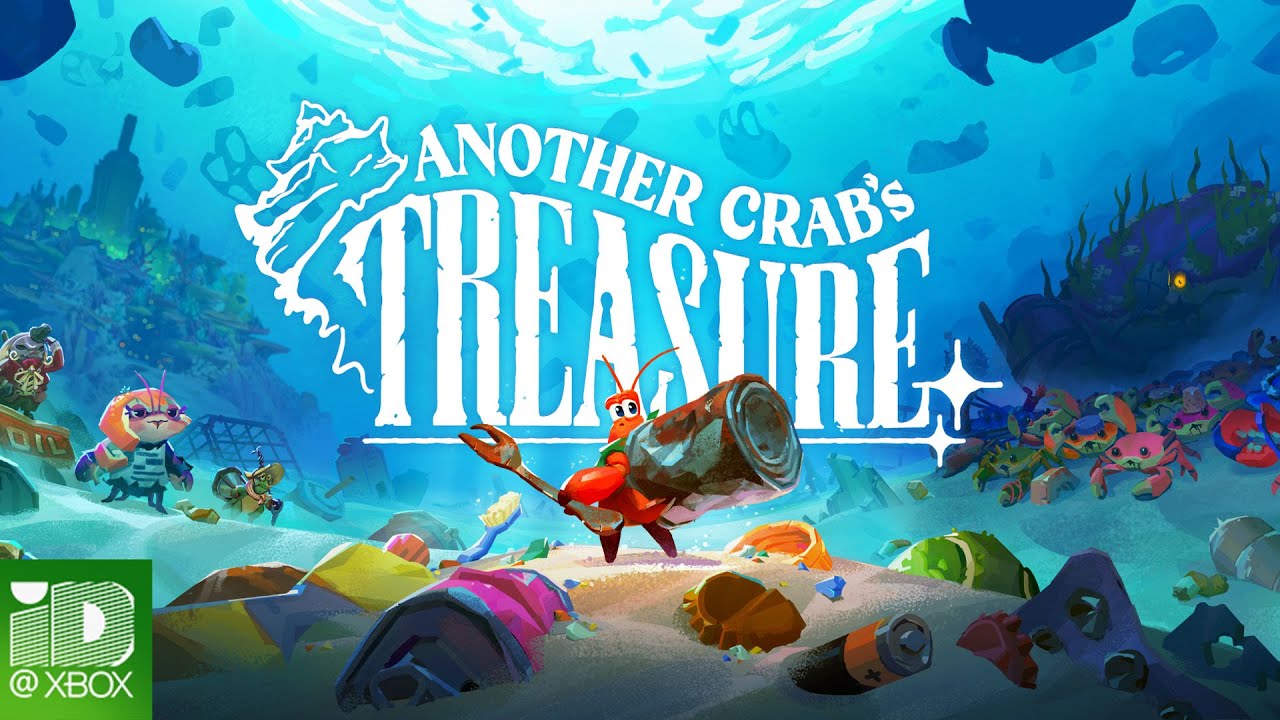The image is a colorful and detailed poster for the video game "Another Crab's Treasure." At the center, a red crab character reminiscent of Sebastian from "The Little Mermaid" wields a two-pronged fork. Instead of a traditional shell, the crab has a rusty can on its back. Surrounding the main character are various other cartoon-like crabs and sea creatures, enhancing the animated underwater setting. The title "Another Crab's Treasure" is prominently displayed in curvy white text, with a seashell accent on the "T" in "Treasure" and a decorative line with two stars underneath. The backdrop features an underwater scene filled with debris and trash, such as an orange pail, a battery, a Bluetooth brush, clothing, and more, illustrating a polluted ocean floor. A hint of a submerged village can also be seen in the background. The bottom left corner of the poster includes the "ID@Xbox" logo, indicating the game's platform.